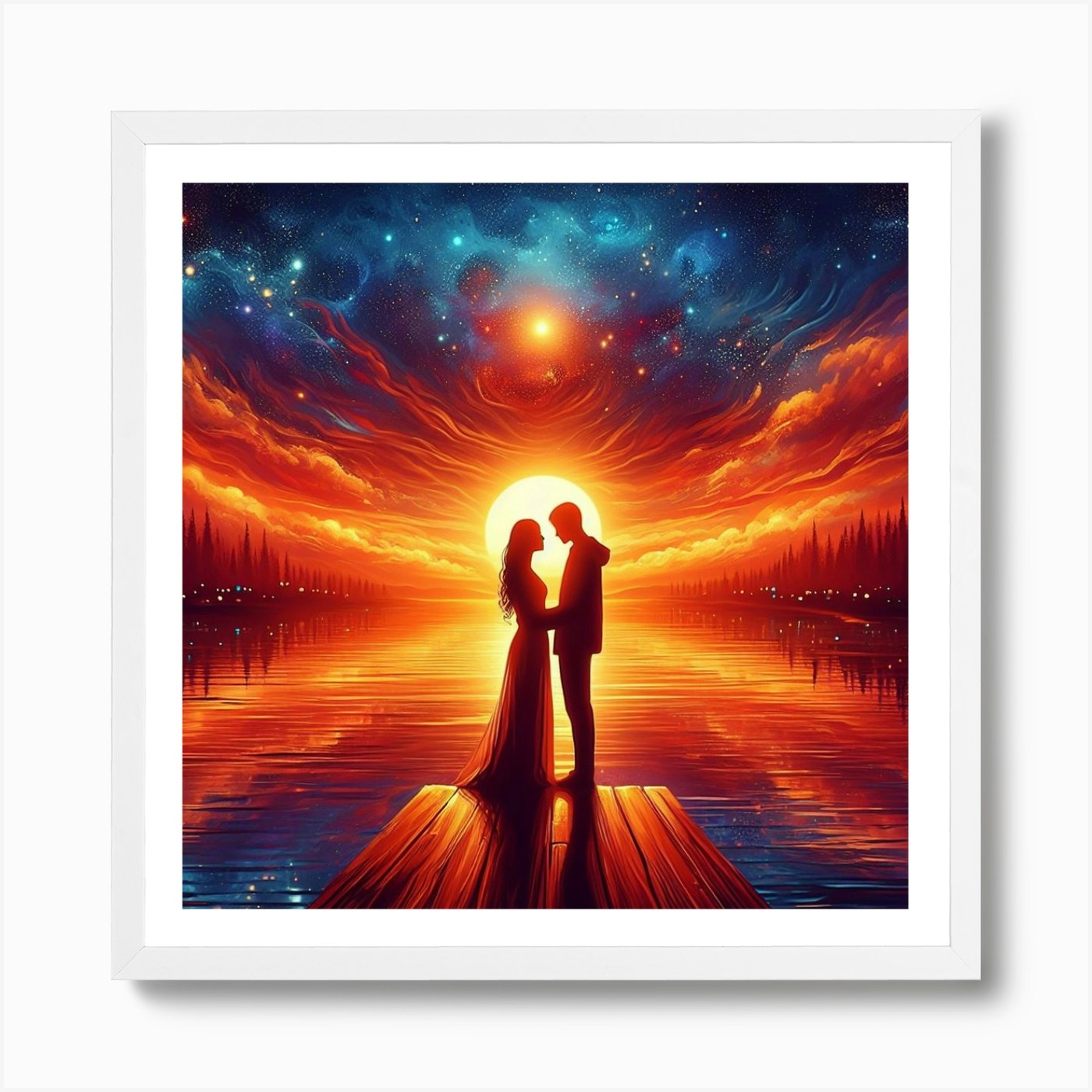The image is an artistic illustration, likely a painting or digital artwork, depicting a silhouetted couple standing on an edge of a dock over the water. The couple, a man in a hoodie and a woman in a dress, are facing each other, holding hands, with the man being slightly taller. They are backlit by a bright, round sun or moon that casts a radiant glow around them, creating a dramatic silhouette effect. The sky is a surreal mix of a vibrant reddish-yellow sunset and a dark blue starry night, with white and yellow stars scattered amidst cloudy areas. The water below reflects this colorful gradient from yellow to red to orange and extends into purple and blue. On either side of the water, a distant horizon includes a treeline and faint city skyline with scattered lights, adding depth to the scene. The overall color palette includes shades of yellow, red, blue, and black, producing a striking and dreamlike atmosphere. The image is presented as a framed photo, complete with a white border and drop shadow, enhancing its artful presentation.